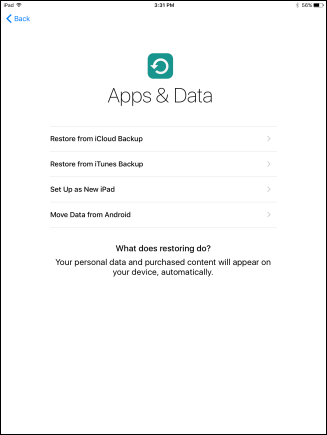The website features a minimalist design, resembling a blank sheet of paper with a white background. At the very top, there is the word "Back" in blue, accompanied by a leftward-pointing arrow. Approximately two inches down from the top, an aqua-green square is prominently displayed. This square features an open circle on its left side and is topped with a triangle-shaped head. Below this icon, "Apps and Data" is written in black letters.

Further down, there are several rectangular buttons each containing black text and grey rightward-pointing arrows. The options available are:
- Restore from iCloud Backup
- Restore from iTunes Backup
- Set Up as New iPad
- Move Data from Android

In the center of the page, a boxed section with a dark black outline contains a message in black text explaining, "What does restoring do? Your personal data and purchased content will appear on your device automatically."